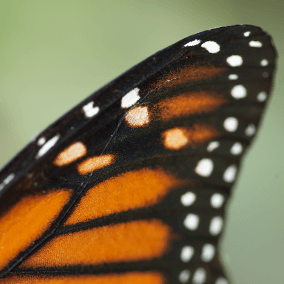This square image captures a close-up view of the wingtip of a monarch butterfly, taken outdoors using natural light. The background is entirely composed of out-of-focus green vegetation, giving an olive-green hue that is slightly more saturated and darker in the upper middle portion. The butterfly’s wing, entering from the bottom left and tapering diagonally toward the top right, dominates the frame. The wing's edges are meticulously trimmed in black, adorned with rows of small white dots—two rows on the right and one on the left. The main body of the wing features a palette of dark, rusty orange with prominent black veins that resemble roots or feather-like patterns. Light plays subtly on the upper portion, adding depth to the tones. Toward the wingtip, the color transitions to black with delicate orange streaks and tiny whitish-yellow circles on top, creating a detailed and intricate visual effect.